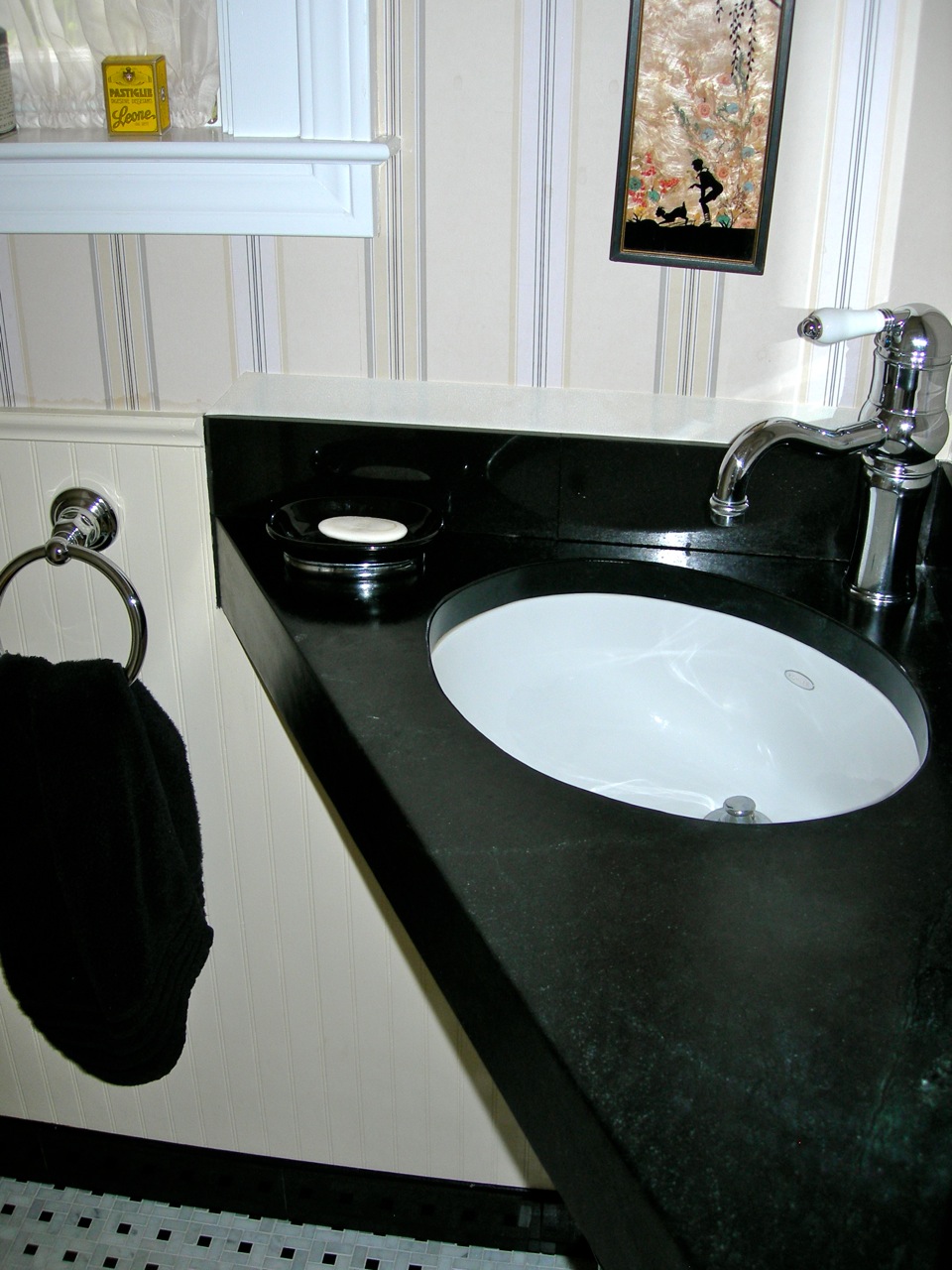The image depicts a cozy bathroom corner featuring a black and white checkered tile floor, barely visible beneath the various elements of the room. The bathroom counter is a sleek, black marble surface with the faucet turned off. Adorning the yellow walls, which have subtle black pinstripes and slightly broader gray stripes, is a piece of decorative art showcasing flowers alongside the silhouettes of a child and a goat, likely crafted from a reflective metal. A towel holder mounted on the wall holds a dark-colored towel, possibly black or very dark brown. Just at the edge of the image is a windowsill with a yellow box perched on it, possibly containing soap or cologne, although the text is unreadable. The corner setup of the sink includes a black soap dish holding a white bar of soap, adding functional elegance to the space.